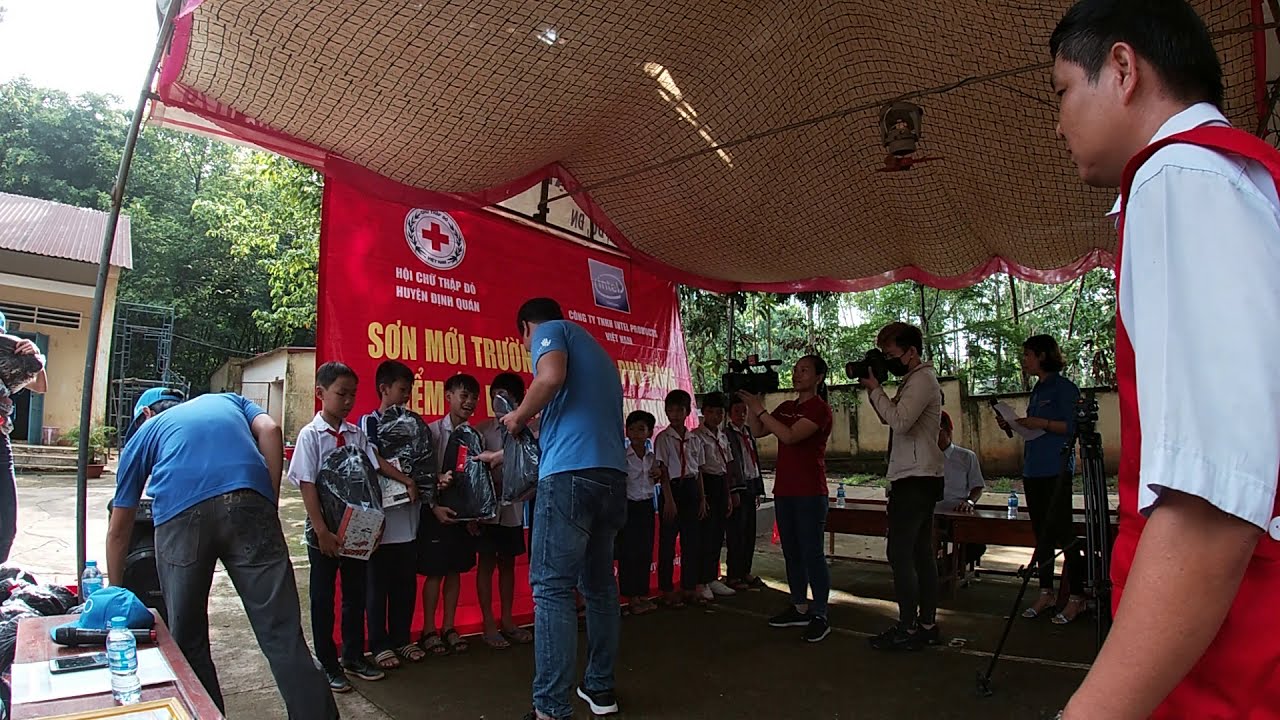This photo captures a group of children, all young boys, standing in uniform comprising white shirts, dark pants, and red ties. They are lined up outside, each holding shiny black objects. The children are standing under a beige canopy, with a large red banner displaying foreign language letters, possibly Thai or Vietnamese, hanging behind them. Surrounding the scene are green trees, indicating it's daytime with tropical foliage in the background. In front of the children are two men wearing blue shirts and jeans; one of them leans toward the left. To the man's left, two people are operating a large camera to photograph the children. On the right side of the image stands another man clad in a red vest and white shirt, observing the scene. It appears this photograph might be capturing a moment from an award ceremony or event where the children are being given bags containing something by the men in front of them.